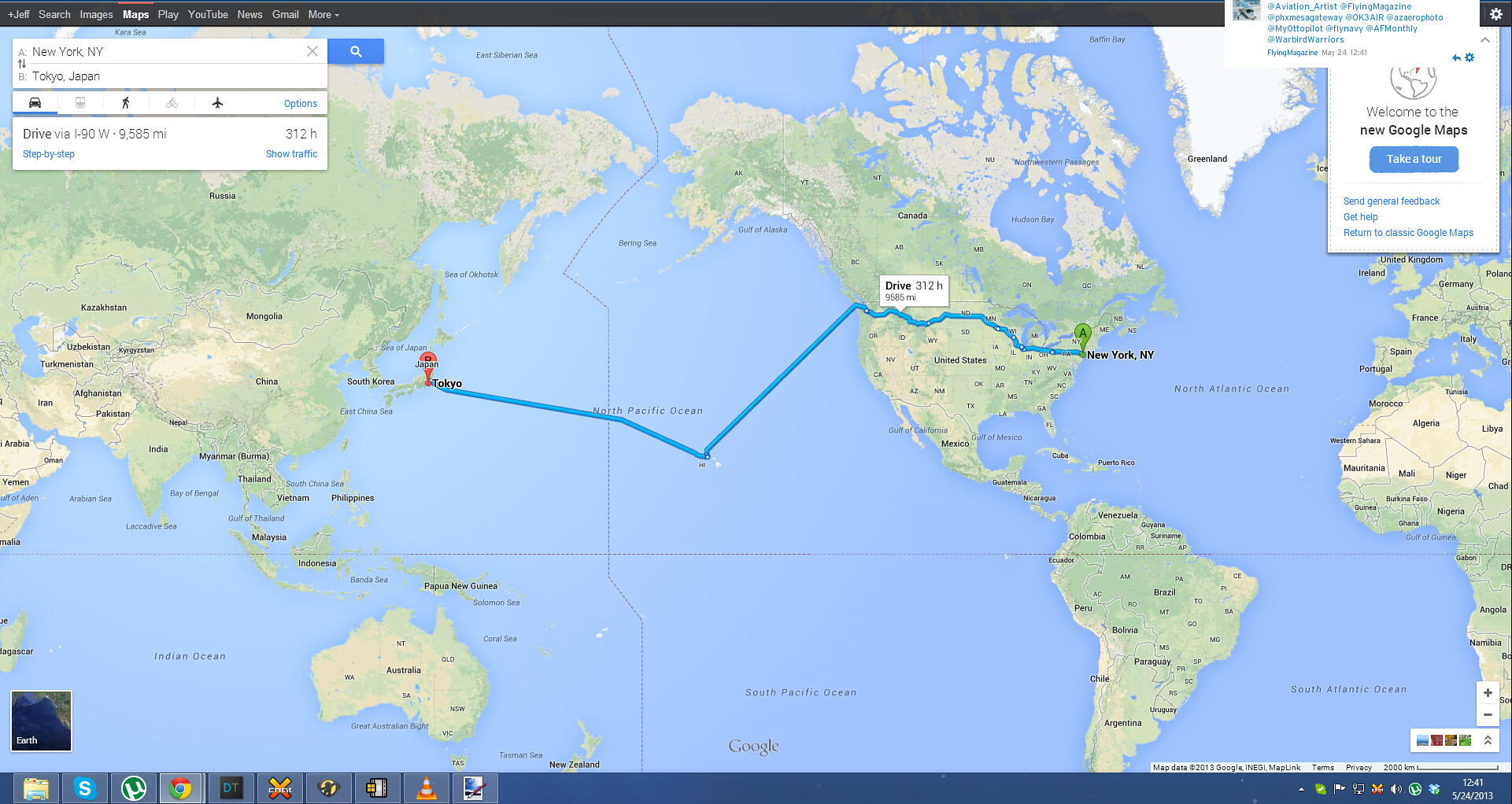The image is a horizontally long, rectangular screenshot of a desktop display, featuring a world map. The map is open on the desktop screen, as evidenced by the bottom toolbar displaying various icons, including a document file, Chrome browser, and a safety cone, indicating it might be VLC media player. The date "5-24-2013" and the time "12:41" are clearly visible in the lower right corner of the screen. 

The world map encompasses all the continents, and prominently features a blue line illustrating a hypothetical journey that starts in New York and ends in Tokyo. The map labels this route as a 312-hour drive. However, this route is impractical for driving due to the vast expanse of the Pacific Ocean separating the two continents.